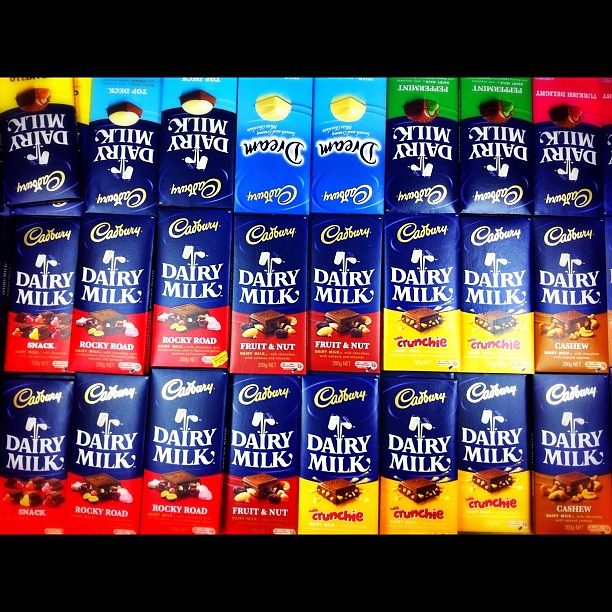The image depicts a neatly arranged display of 24 Cadbury Dairy Milk Chocolate Bars, showcasing a variety of flavors. Each bar features the iconic Cadbury logo set against the brand's signature blue background. The lower portion of each packaging varies in color—red, yellow, or green—indicating the specific type of bar. Among the recognizable flavors are rocky road, fruit and nut, crunchy, cashew, peppermint, and top deck. Additionally, there is a bar labeled "Dream" and another with upside-down text, making it difficult to read. All the bars are lined up in rows against a black background, bordered at the top and bottom to emphasize the array of colorful packaging. A glass of milk with milk pouring out is also visible, reinforcing the Dairy Milk branding.